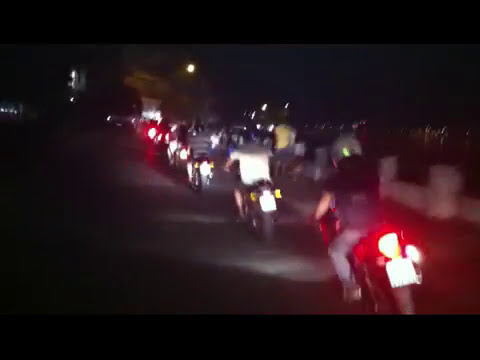In this low-quality photograph, a group of approximately ten motorcycles is seen riding single file along a dark street at night. The scene is enveloped in darkness, with black borders framing the image. The riders, some paired and others riding solo, are dressed in t-shirts and shorts, indicating a warmer climate. The motorcycles' red and white taillights create a bright contrast against the night. To the right of the riders, there is a white structure, possibly a fence, and the faint outline of pedestrians overlooking what might be water. In the far background, city lights glimmer faintly. The last rider in line is identifiable by a green helmet, blue jeans, and a dark shirt, while the rider in front of him wears a white shirt and black helmet. The person ahead of them sports a striped dark shirt. The entire scene conveys a sense of nighttime adventure, with the motorcycles heading towards an unknown destination.